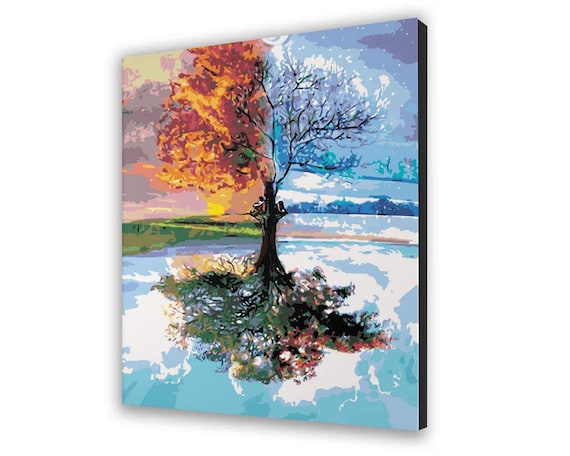The image is a detailed and vibrant artwork depicting a surreal tree that represents all four seasons, set against a stark white background with a shadow around the square-shaped piece. The illustrative style is highly abstract and not realistic. The top left quadrant represents autumn, with the tree adorned in brilliant reds, yellows, and oranges, standing against a purple sky. The surrounding landscape showcases varying shades of green and brown. The top right quadrant depicts winter; the tree is barren, decorated with white snow, and framed by a cloudy, snow-filled sky, with a landscape featuring shades of blue including mountains or houses blanketed in snow. The bottom right represents spring, where the tree starts to bloom with new leaves and vibrant flowers under a cloudy and stormy sky. The grass remains brown, hinting at the receding winter. The bottom left quadrant illustrates summer, displaying a lush, full-canopied tree under partially cloudy skies with very green grass. The tree spans all four sections seamlessly, with each season meticulously illustrated to blend into the next, creating a cohesive representation of the passage of time and nature’s cyclical beauty.